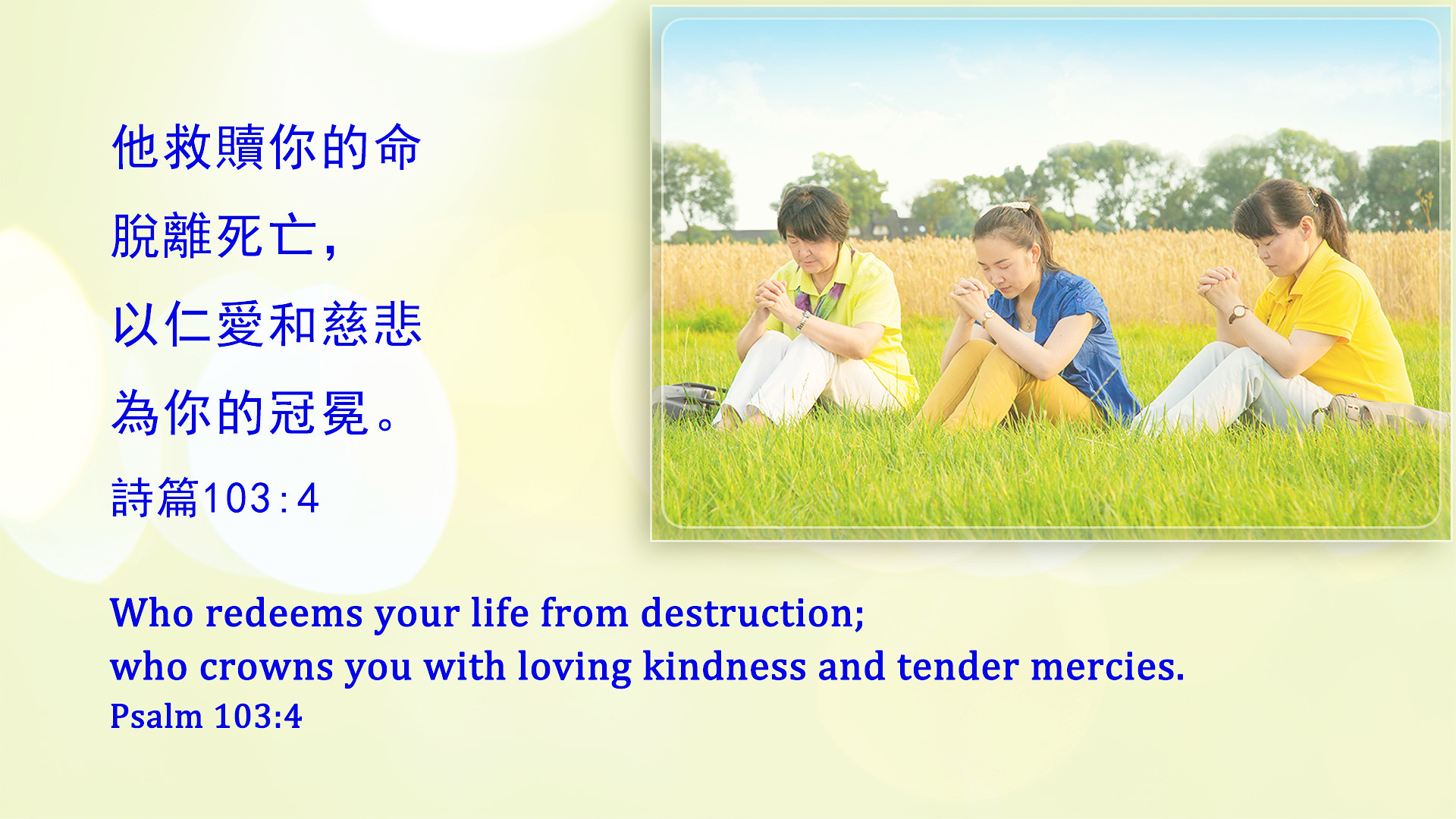This image features a professionally taken photograph set within a pale yellow background adorned with blue Chinese characters and the Bible verse, "Who redeems your life from destruction? Who crowns you with loving kindness and tender mercies? Psalm 103:4," both in Chinese and English text. The photograph depicts three women, likely of different ages, sitting in a lush, green grassy field with their hands clasped in front of them and heads bowed in prayerful reflection. The grassy field transitions to a backdrop of tall, brown grass and distant green trees under a bright blue sky. The woman on the left, who has short brown hair, is dressed in white pants, a yellow collared short-sleeve shirt, and a green and purple scarf, with a bag placed beside her. The middle woman, appearing younger, wears a blue short-sleeved shirt and yellow pants, hair pulled back into a ponytail. The woman on the right, also with hair in a ponytail, is dressed in a yellow shirt and white pants, and sports a wristwatch.